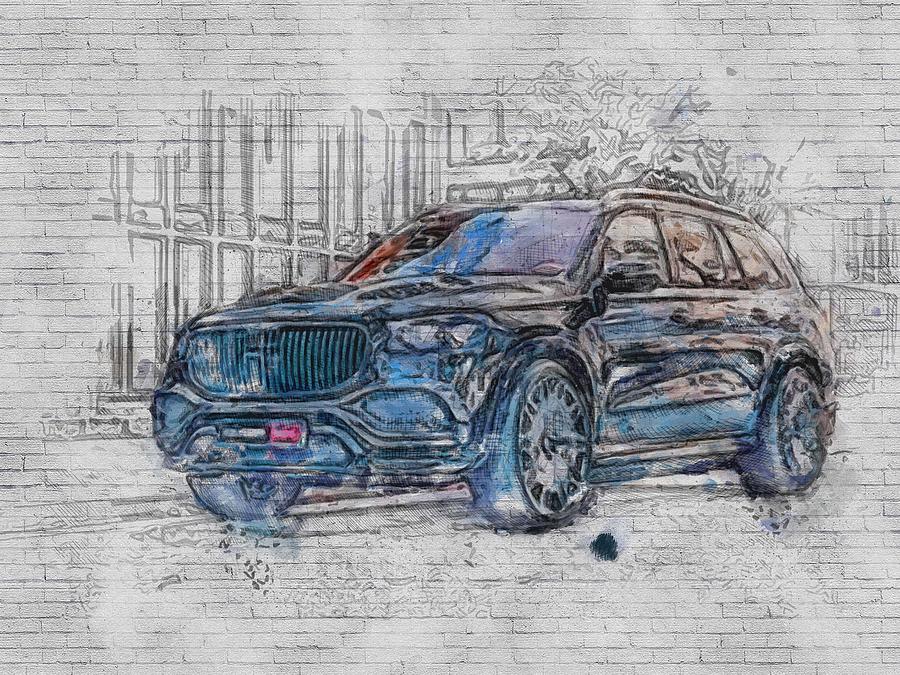The image depicts an embossed painting set against a slightly weathered white brick backdrop. The main focus is a detailed blue SUV, accentuated with black outlines and touches of red, pink, and brown to add depth. The SUV has a grill with an 'H' emblem, large tires, and three brownish windows on the visible side, though the interior details remain obscured. The vehicle is depicted facing left, emerging from the wall as if in motion, with three wheels visible. Additional details include a red and black license plate area below the grill and a luggage rack on top. The faint outlines of buildings, windows, and a tree subtly enhance the background scenery.